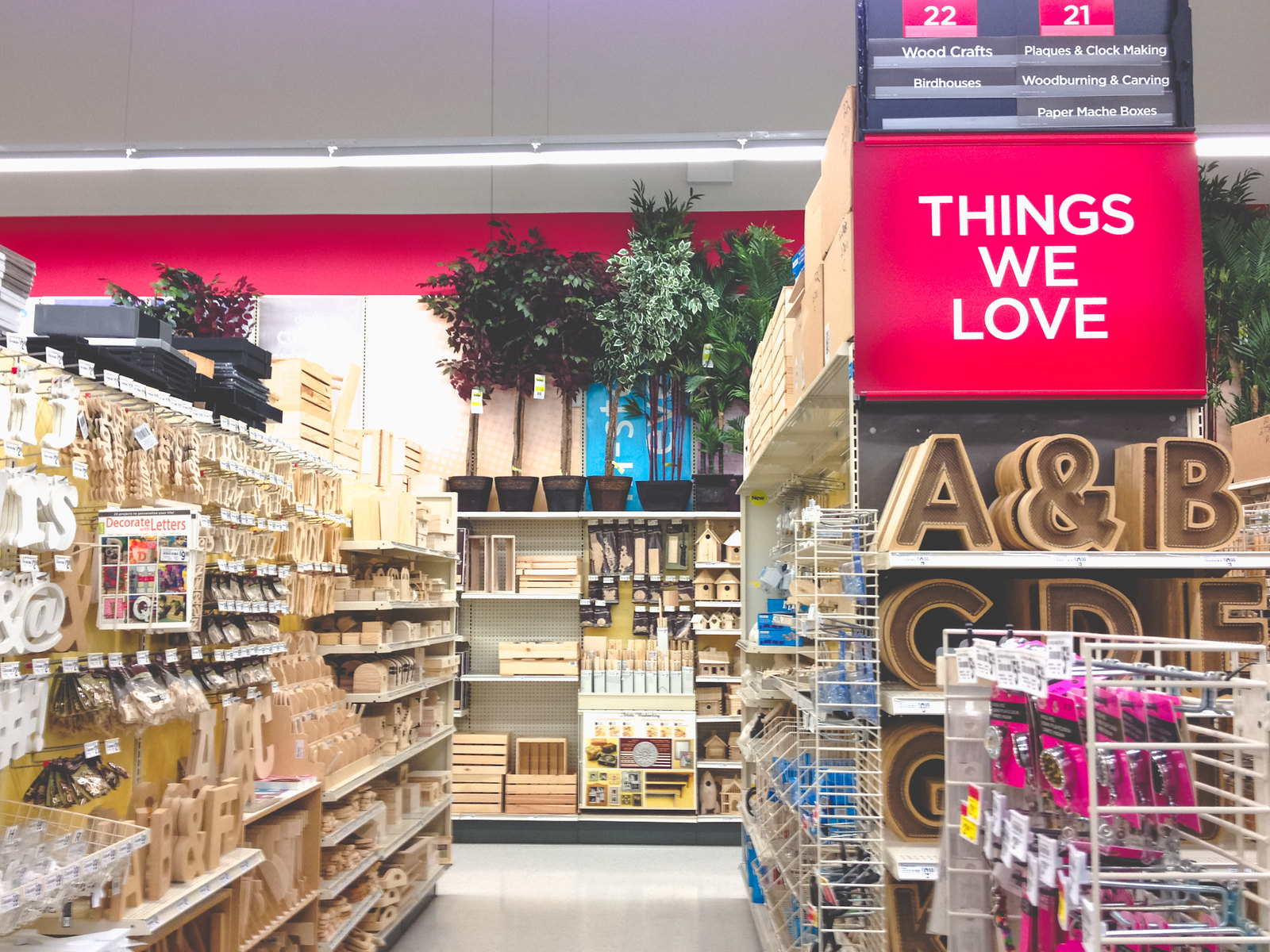Inside a retail craft store, an aisle marked with a vibrant hot pink sign—emblazoned with the playful phrase "Things We Love" in crisp white font—draws attention. Flanking the sign, Aisle 22 on the left features an array of woodcraft materials and intricately designed birdhouses. On the right, Aisle 21 is dedicated to plaques, clockmaking supplies, wood burning and carving tools, and a selection of paper mache boxes. The end cap near the sign is adorned with wooden alphabet letters and an ampersand, inviting creativity. Beyond this display, an assortment of artificial floor plants is visible, enhancing the store's vibrant and resourceful ambiance. Everywhere, shelves brim with wooden craft items, showcasing the extensive range of creative supplies the store offers. The scene, whether real or computer-generated, immerses one in a haven for craft enthusiasts.